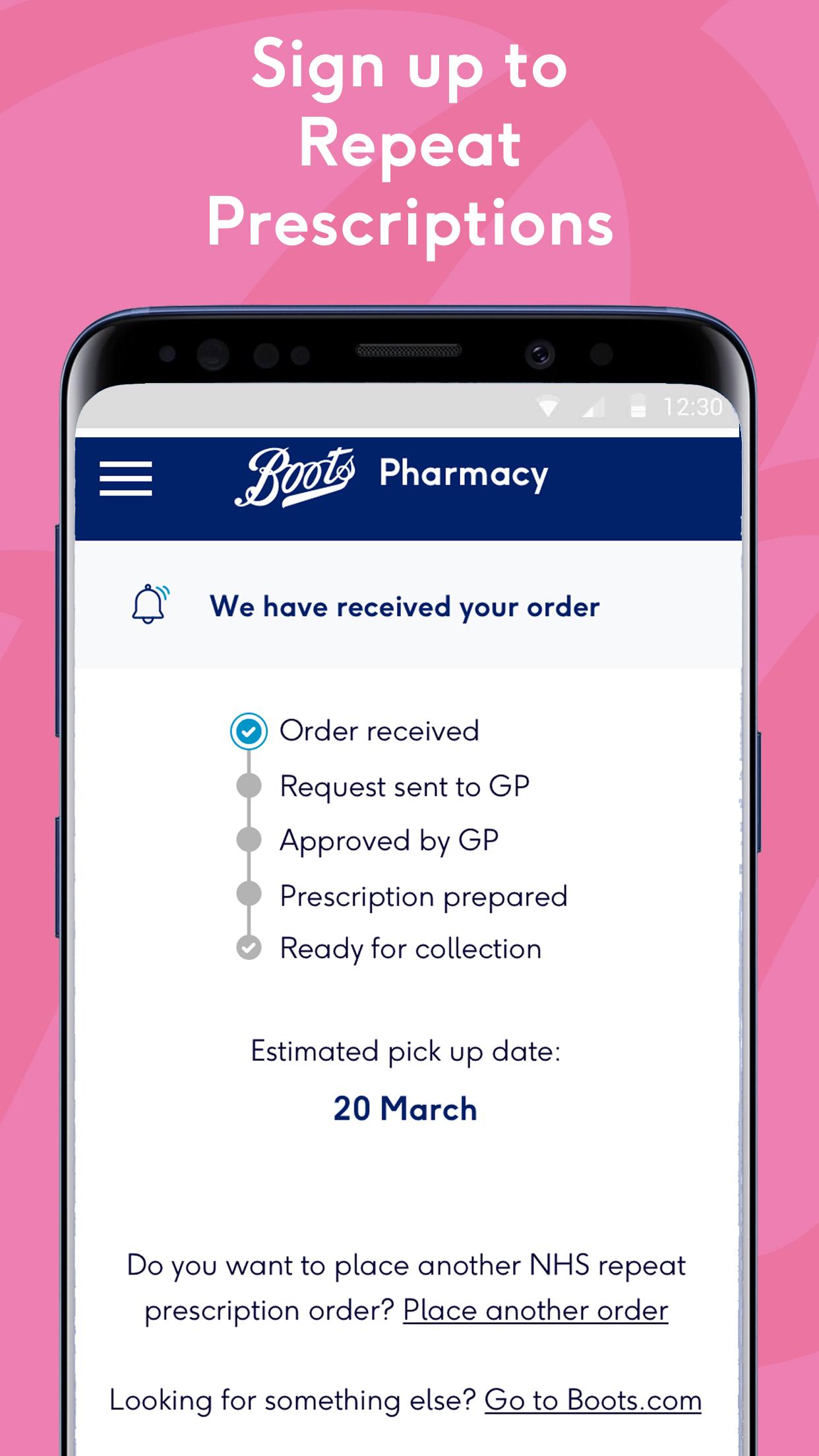The vertical image seems to be a screenshot from an advertisement. The background features varying shades of pink, with a dark, almost sorely pink at the top blending into a slightly lighter mauvey pink beneath it. At the bottom, the image abruptly cuts off into the white background of a computer screen.

In bold white text at the top of the image, it says, "Sign up to repeat prescriptions." Below this text, there is an image of a smartphone with a black rim. The smartphone display includes a gray status bar with typical icons, such as a downward-pointing triangle, signal strength indicator, battery life, and the time displayed as 12:30. A black section at the top houses the camera.

Within the smartphone screen, there's a blue box with white text that reads "Boots Pharmacy." Beneath this, a lighter gray box contains the message, "We have received your order," accompanied by a small bell icon. The interface presents a chronological process with the following stages: Order Received, Request to GP, Approved by GP, Prescription Prepared, Ready for Collection, and Estimated Pickup. The estimated pickup date is highlighted in blue as the 20th of March.

At the bottom of the smartphone screen, there are options to "Place another NHS repeat prescription order," "Place another order," "Look for something else," or "Go to boots.com." Buttons are available to place another order or navigate to boots.com.